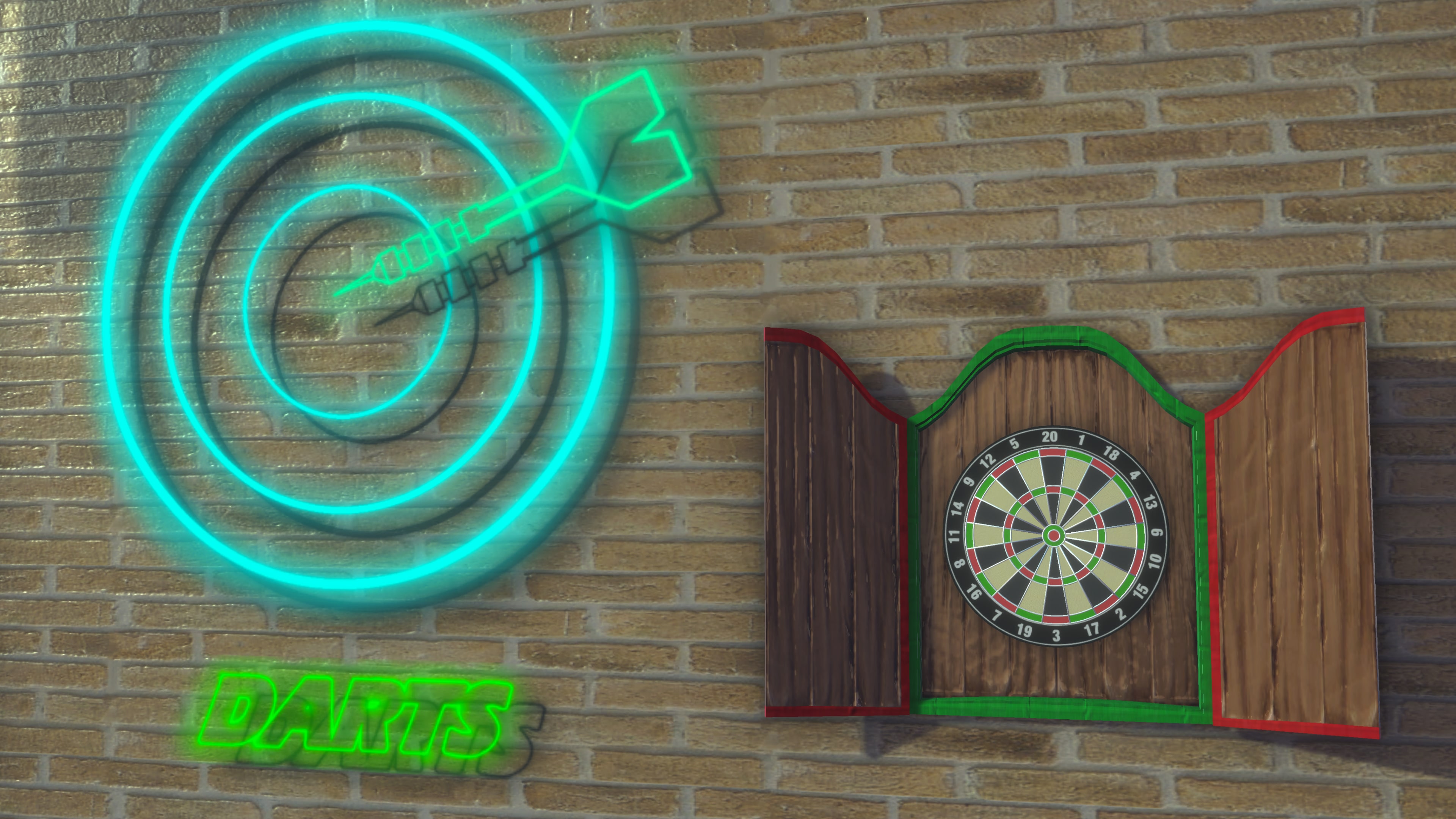The photograph captures an interior red brick wall adorned with two focal decorations. On the right side of the wall, there is a rustic, distressed wooden cabinet with doors outlined in red and green trim that houses a traditional dartboard. The dartboard features a black outer ring, white numbers, and alternating colors of cream, red, green, and black. To the left of this cabinet, a vibrant neon sign stands out. The sign features concentric circles in a light blue, mimicking the layout of a dartboard, with a prominent neon green dart pointing towards the center. Below this, "darts" is spelled out in lime green neon letters, adding a playful and dynamic touch to the brick wall.